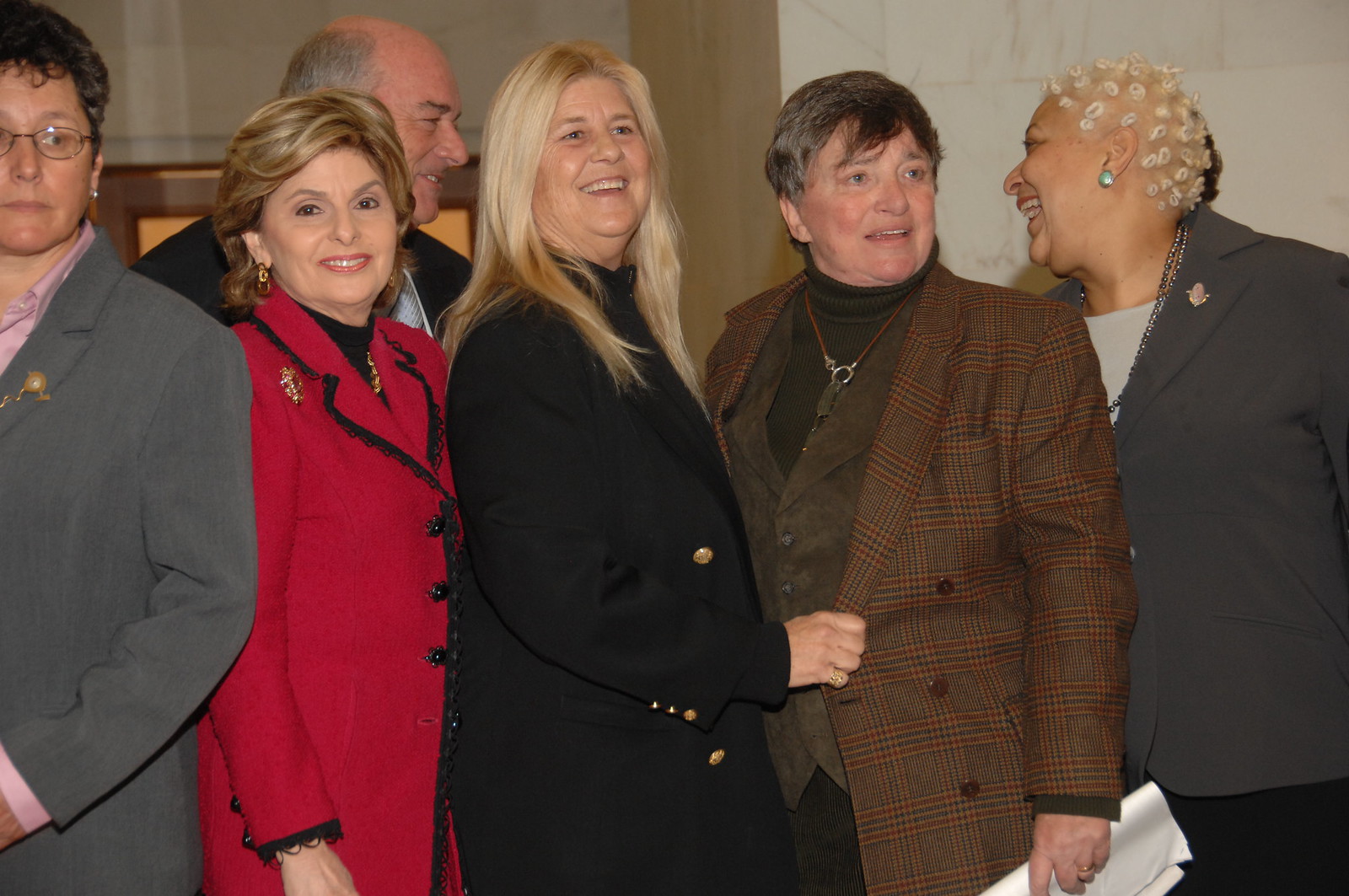In the center of this indoor image, six individuals are posing in front of a light marble stone wall, punctuated by a column where the walls converge. The group appears to be dressed in business attire suitable for a wintertime office environment. At the forefront, a woman in a red coat jacket looks directly at the camera. To her left, another woman in a black long coat with blonde hair smiles while holding a brown plaid coat belonging to a woman beside her, who clutches papers. On the right, a woman with unique blonde hair styled in what appear to be bumps is dressed in a blue dress coat, looking away from the camera. Behind them stands a balding man in a black suit jacket, engaged in conversation with a woman in a gray jacket on the far right. Another woman in a gray suit, slightly to the left, also looks away from the camera. There is an indistinct sign and some glass elements partially obstructed by the group. The image lacks visible text, and the predominant colors include gray, tan, brown, red, green, black, and white. Multiple people taking photos can be inferred due to differing gaze directions among the group members.